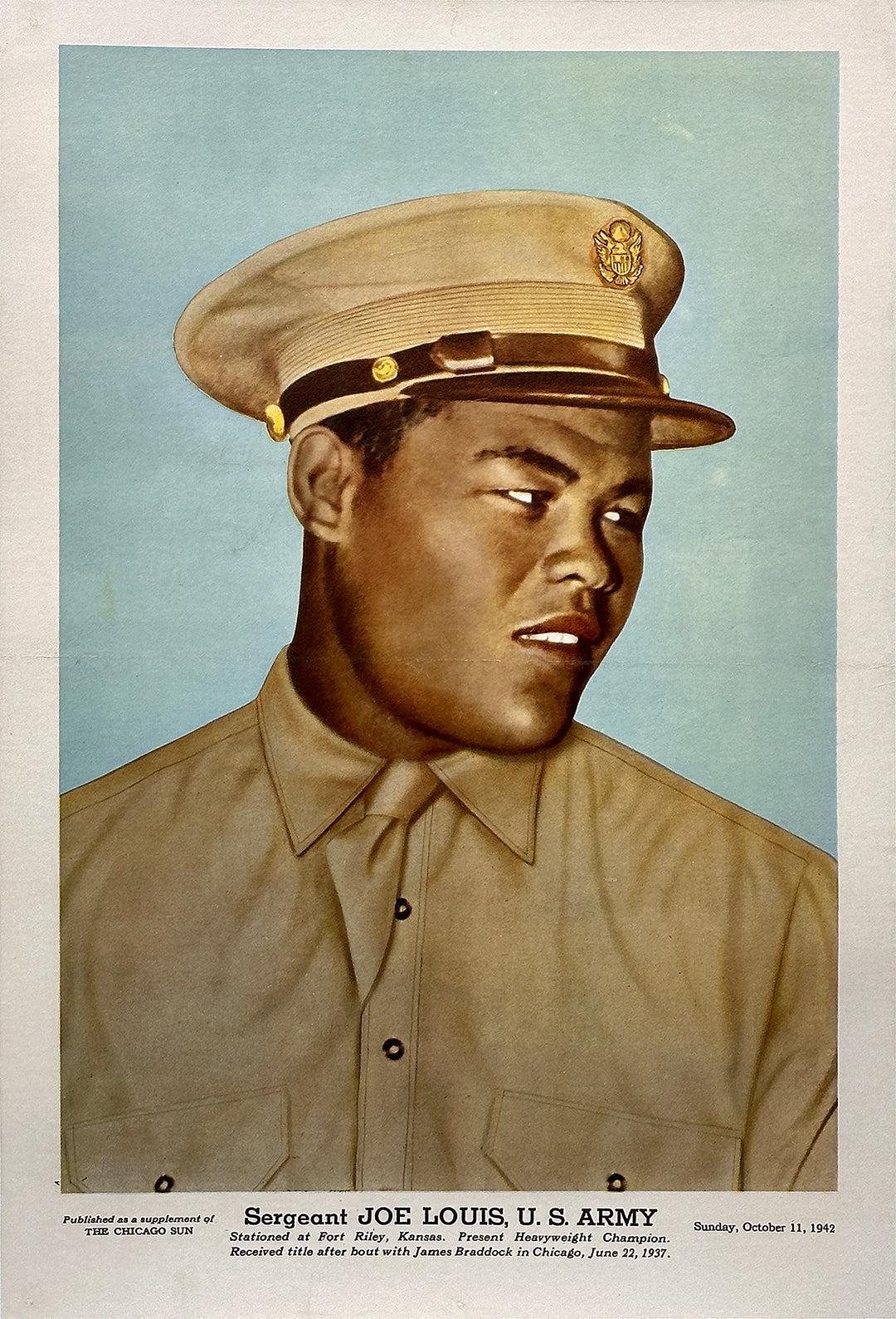The image features an African American soldier wearing a military uniform. The soldier is donning a formal military-style hat adorned with a gold emblem at the top, a black band accented with gold buttons, and a black brim. He is captured in profile, gazing to the side with a somber or concerned expression. His attire includes a beige shirt. Below the image, text identifies him as Sergeant Joe Lewis of the U.S. Army, stationed at Port Riley, Kansas. It notes that he is the present heavyweight champion and mentions his bout with James Braddock in Chicago on June 22, 1937. Additional text to the right of this main information reads, "Sunday, October 11, 1942." To the left of the main text block, it is noted that the image was published in a supplement to the Chicago Sun.